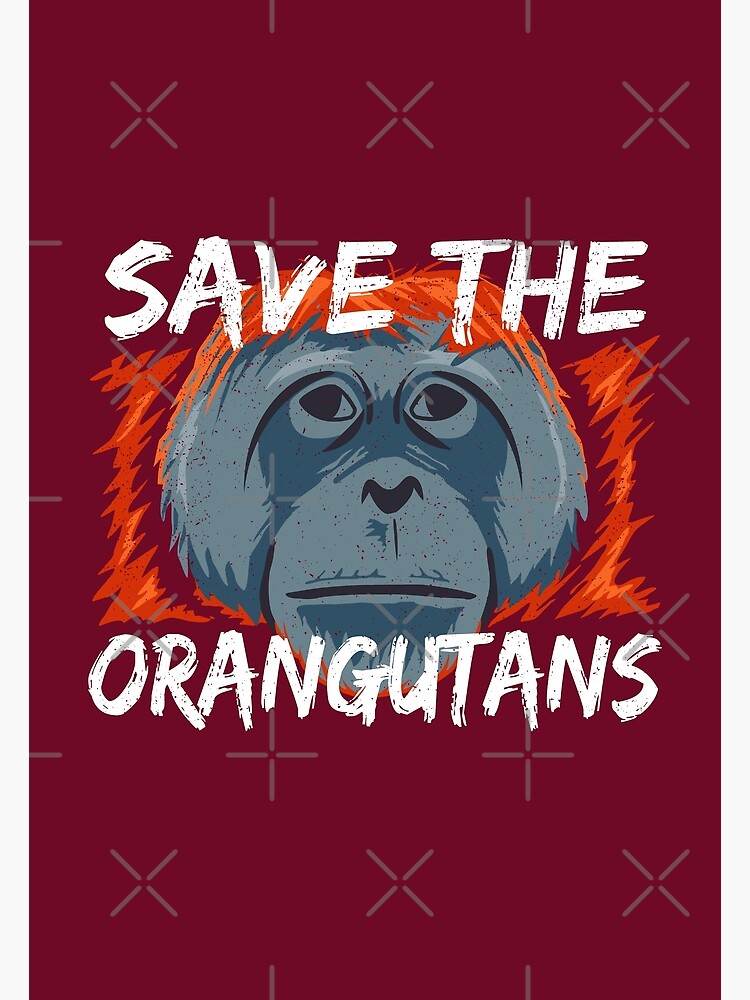This poster features a digitally created or hand-drawn graphic design with a bold and vivid visual style. The background is a rich, pinkish-red hue, veering towards a deep brick red, adorned with a repeating pattern of grayish white X's and crosses. Central to the composition is a striking depiction of an orangutan's face. The orangutan, rendered with a lineless art style, has a gray face with realistic proportions, though its eyes appear to be looking in different directions, conveying a solemn expression. The orangutan's head is surrounded by scratchy orange fur, which is highlighted with darker orange shading. Prominently overlaying the image in a chalk-like, sketchy white script are the words "SAVE THE" across the orangutan's forehead and "ORANGUTANS" right below its chin. The text, along with the background pattern and the detailed portrayal of the orangutan, create a compelling and heartfelt appeal to save these endangered creatures.